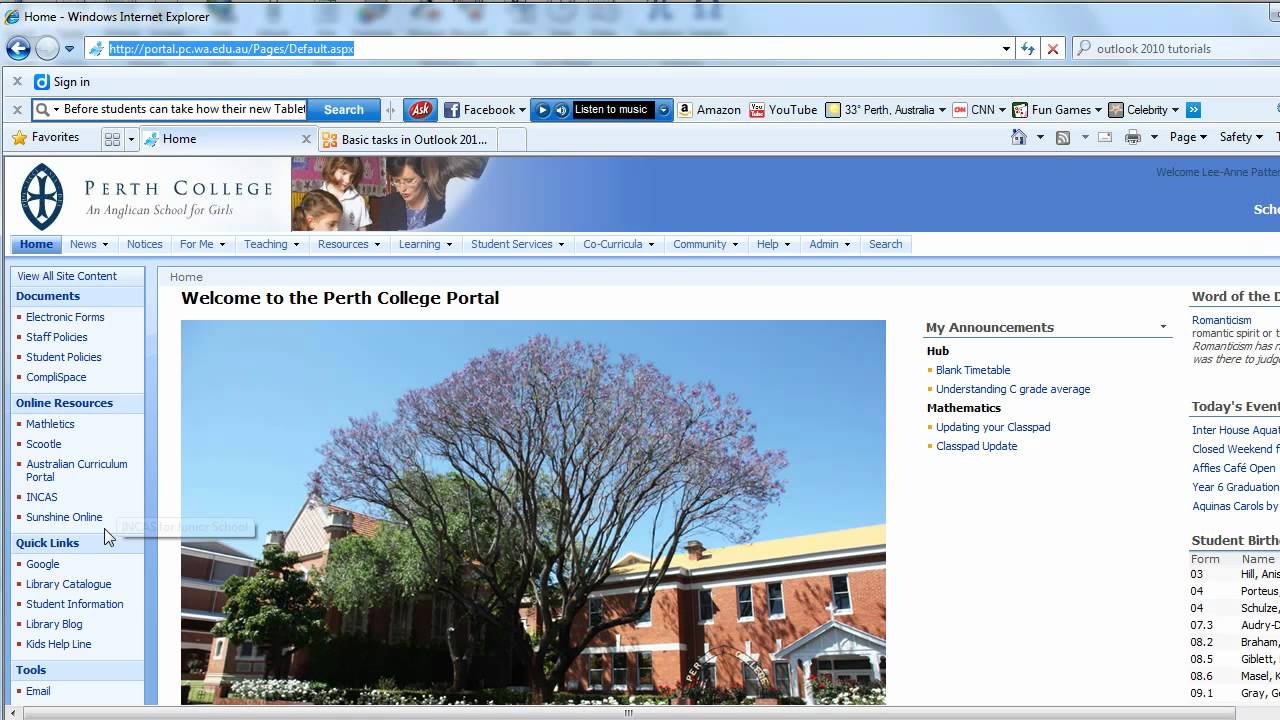This is a detailed screenshot from a college website, captured from an old version of Windows Internet Explorer. The webpage belongs to Perth College, an Anglican school for girls. In the navigation bar at the top, there is a small image depicting an adult woman with glasses, short hair, wearing a blue jacket and shirt, engaged in a conversation with three children. 

The main section of the webpage is titled "Welcome to the Perth College Portal" and features an image of the college itself. The campus picture showcases a prominent sign that reads "Perth College," surrounded by neatly arranged red and white flowers. Multiple trees adorn the scene, with the largest tree boasting vibrant purple flowers, while the smaller ones are lush with green leaves. The backdrop is a clear blue sky, providing a serene atmosphere.

To the right of the campus image, various options are listed, including "My Announcements," "Hub," "Blank Timetable," "Understanding C Grade Average," "Mathematics," "Updating Your ClassPad," and "ClassPad Update." On the left side of the screen, a panel offers links to "View All Site Content," "Documents," "Online Resources," "Quick Links," and "Tools."

At the very top of the browser window, you can see multiple tabs open, including Amazon, Facebook, YouTube, CNN, Fun Games, and Celebrity.